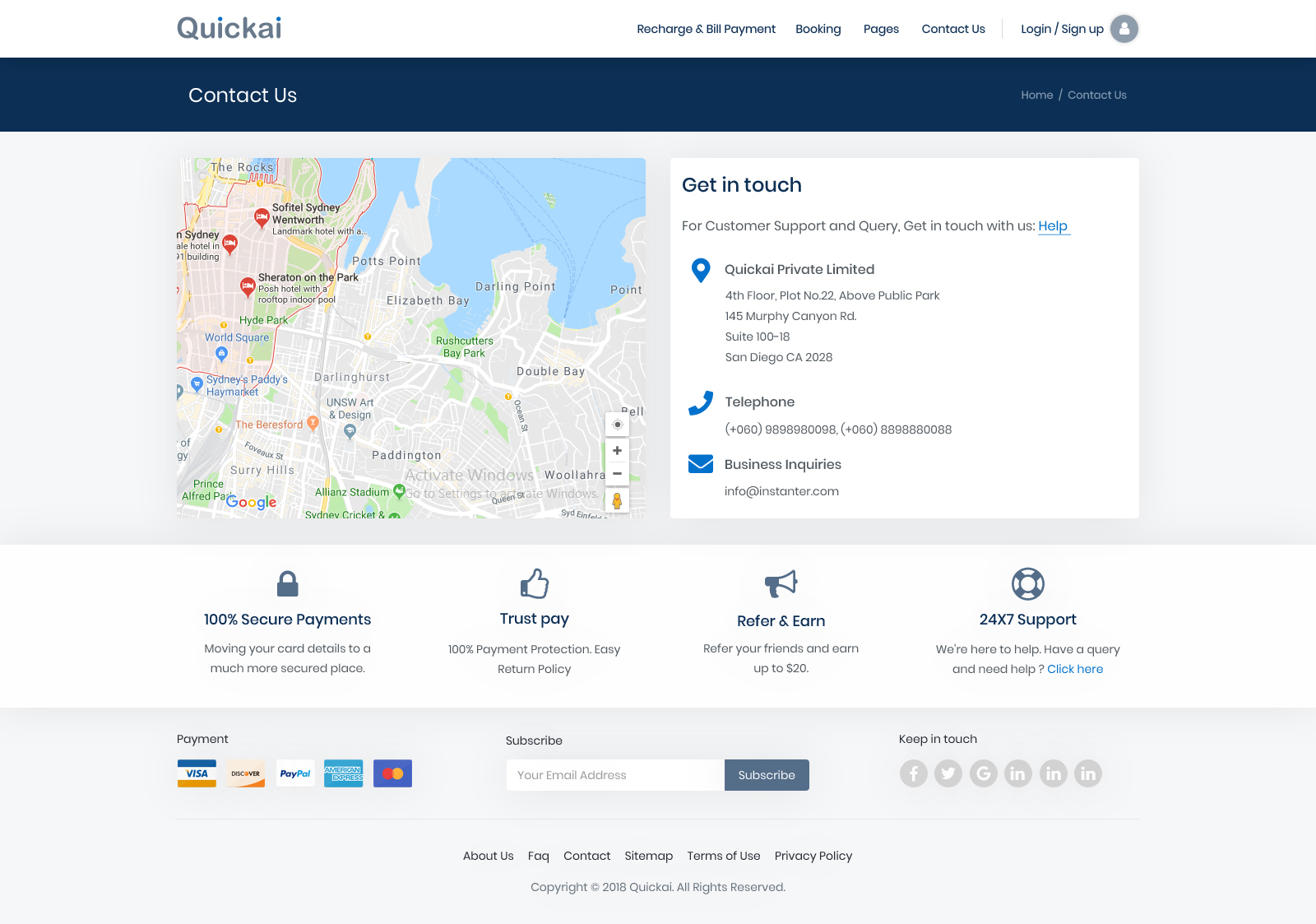The image displays a computer screenshot of an advertisement for a website titled "QuickAI" in the top-left corner. In the upper section, a blue-black bar features a "Contact Us" link. Below this, a detailed map showcases several areas, including Sofitel Sydney Wentworth, Hyde Park, Sydney's Paddy’s Haymarket, and Surrey Hills, with a body of water positioned at the top of the map.

On the right side, there is a small white box with the heading "Get in Touch." The text below encourages users to contact them for customer support and queries, highlighting a "Help" button. This section identifies the company as "QuickATI Private Limited," based in San Diego, California, and provides a telephone number and an email address for contact.

Beneath this information, a white bar displays icons and text promoting various service guarantees. A lock symbol indicates "100% Secure Payments," and a thumbs up symbol notes "Trust Pay," which ensures 100% payment protection and an easy return policy. A megaphone symbol emphasizes a "Refer and Earn" program, offering users up to $20 for referrals. Another symbol mentions 24/7 support availability.

At the bottom, a gray box outlines payment methods and includes a space for subscribing, enhancing the user experience with comprehensive options for engagement and support.